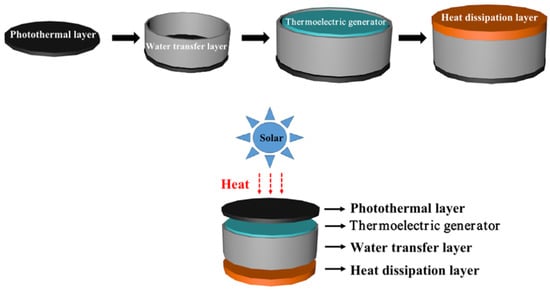This scientific illustration utilizes computer-generated graphics to depict the structure and function of a multi-layered thermoelectric generator designed for solar heat conversion. At the forefront of the diagram sits a representation of the sun, labeled "solar," radiating blue light with three red arrows labeled "heat" descending towards the device. The device itself is shown in an exploded view, revealing each of its four functional layers stacked from top to bottom.

The topmost layer is the photothermal layer, depicted as black and flat, which directly absorbs sunlight and converts it into heat. Beneath it lies the water transfer layer, illustrated in a silver color, responsible for transferring the heat generated. The third layer is the thermoelectric generator, shown in a bluish-green hue, which converts the transferred thermal energy into electrical energy. Lastly, the bottommost layer is the heat dissipation layer, depicted in orange, which releases any excess heat from the system.

Each layer is clearly labeled and displayed both in their stacked configuration and in an exploded view with arrows illustrating their interactions, emphasizing the device's function of converting solar energy into usable heat and electricity. The overall colors of the illustration include silver, black, white, and touches of blue, supporting the scientific and technological aesthetic, with prominent labeling to help identify each critical component.